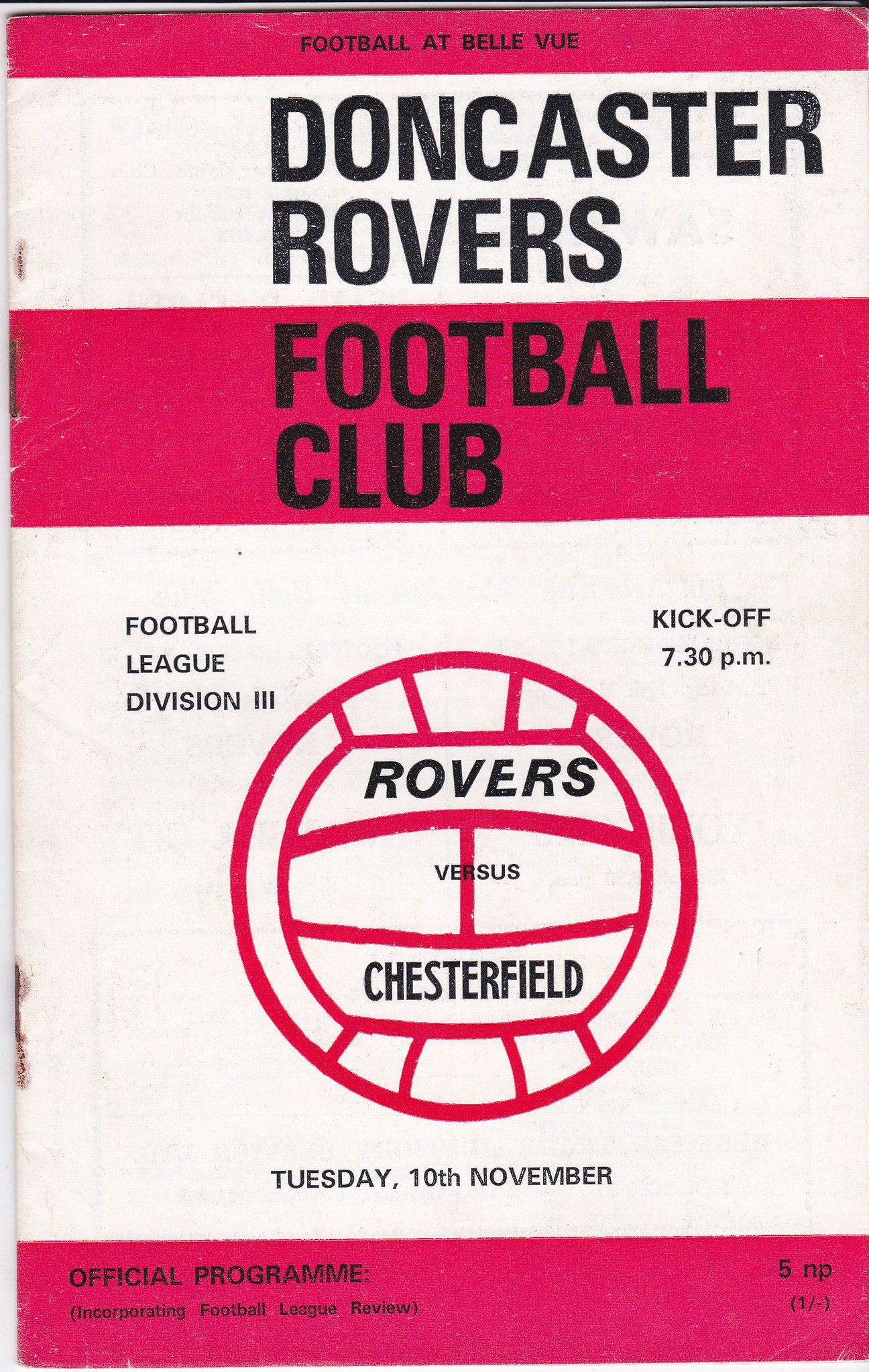This is an image of an older football program cover for a match featuring Doncaster Rovers Football Club. The cover is designed with horizontal red and white stripes, with a prominent red stripe at the top. At the very top, in black text, it reads "Football at Bellevue". Beneath this, there is a white stripe with the text "Doncaster Rovers Football Club" in black. In the center of the cover, there is an outline of a soccer ball. Around this ball graphic, it states "Rovers versus Chesterfield" and "Football League Division Three" in black text. To the right of the ball graphic, it notes the kickoff time as "7.30 p.m." Below the ball, the date is printed as "Tuesday 10th November". The bottom of the cover is bordered with red and includes additional text in the left-hand corner: "Official Program Incorporating Football League Review". In the same corner, it also lists the price as "5p" with peculiar formatting including "1/-" and parentheses around "p". The overall condition of the program suggests age, and it appears to be bound with staples with some visible damage to the border.